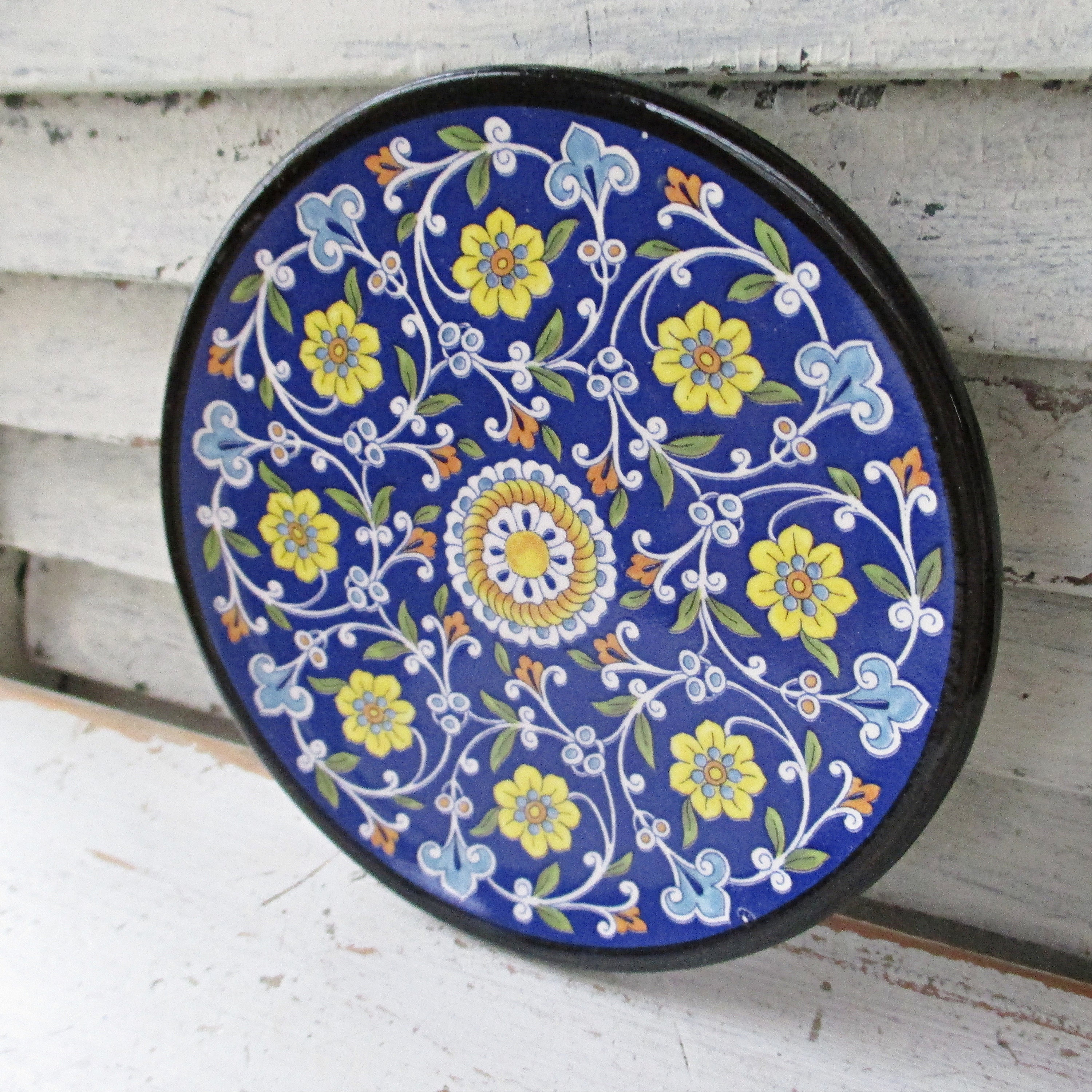This photograph was taken outdoors and prominently features a blue, floral-patterned plate, possibly a trivet, leaning against the white, chipped-painted wooden siding of a house. The plate, in excellent condition and quite shiny, has a detailed design with a large yellow flower at its center, surrounded by smaller yellow, blue, and orange flowers, all encircled by white vines with green leaves. The black-rimmed plate sits on a worn white wooden table, with visible wood peeking through the chipped paint. The white siding behind the plate is horizontal slats, extending four rows high, and sits above what appears to be a cement foundation.